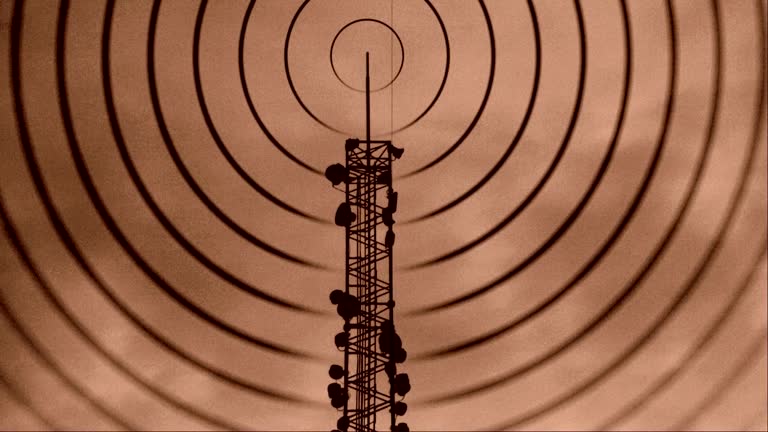This image features the top segment of a cell tower, structured like an erector set, set against a sepia-toned backdrop with shades of brown, dark brown, and hints of orange and white, reminiscent of a lightly stormy or cloudy day. The tower rises prominently from the bottom center, extending upwards. Along its sides, various antenna dishes and speakers, silhouetted in black, are attached, suggesting the transmission of different signals. The uppermost point of the tower holds a tall, thin antenna, encircled by seven concentric rings. These rings, sketched in black and gradually decreasing in size towards the top, visually represent the radio frequency waves emitted from the antenna, akin to a bullseye pattern. The stark image captivates with its minimalism and the intricate details of the tower structure and frequency visualization.